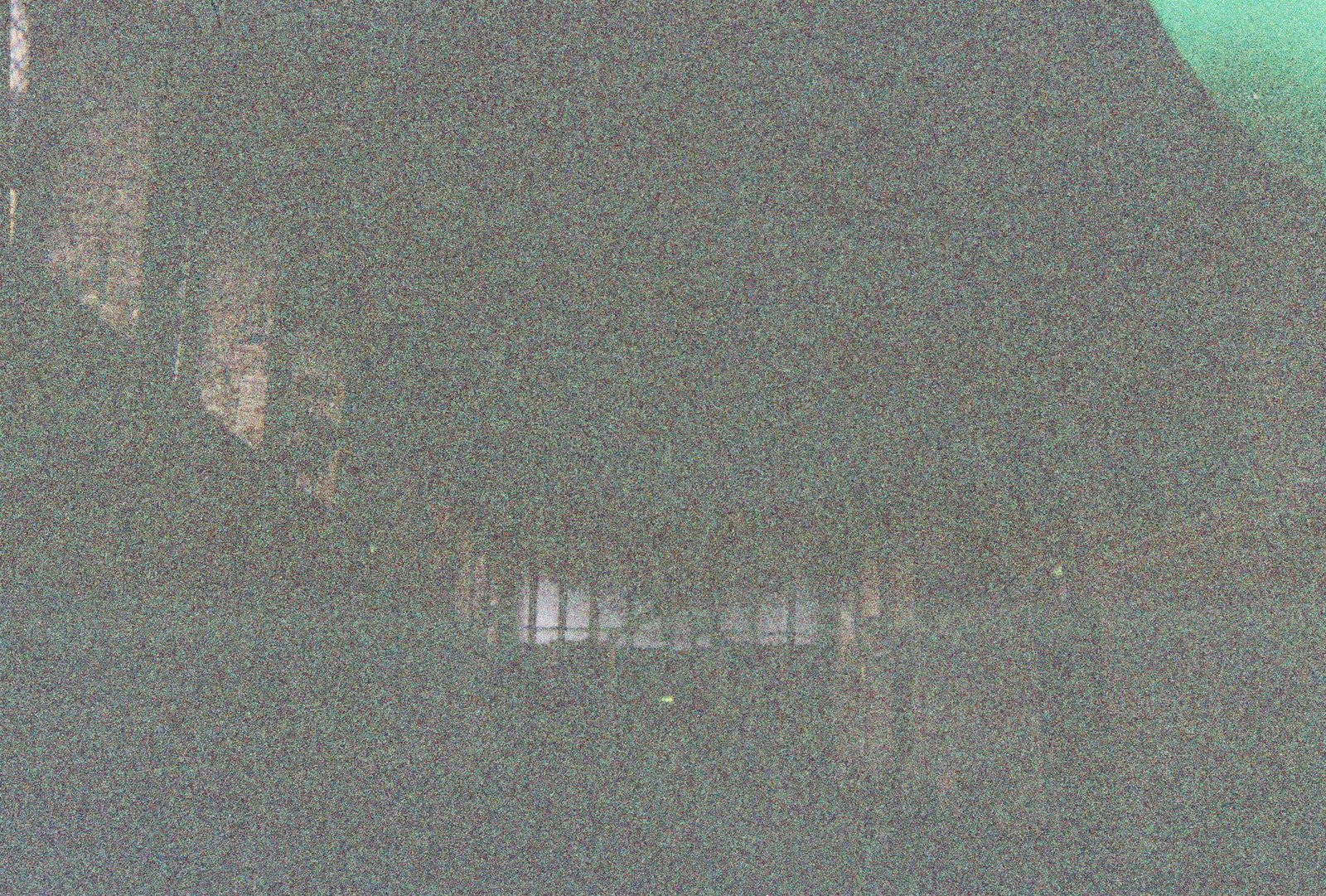In this washed-out and blurry photograph, a large indoor space, potentially a warehouse or a bus or train station, is depicted. The overall image has a heavy grainy texture. Dominating the central perspective is a row of windows, through which light softly filters into the scene. On the left side of the image, three windows, possibly embedded into brick walls, further emphasize the architectural details of the structure. The visible areas of the building indicate a color palette of reds, tans, and browns, suggesting the use of brick in its construction. In the upper right corner, a large, green, circular distortion is noticeable, likely a flaw or artifact within the image itself. The combination of these elements strongly suggests that the photograph was taken indoors.